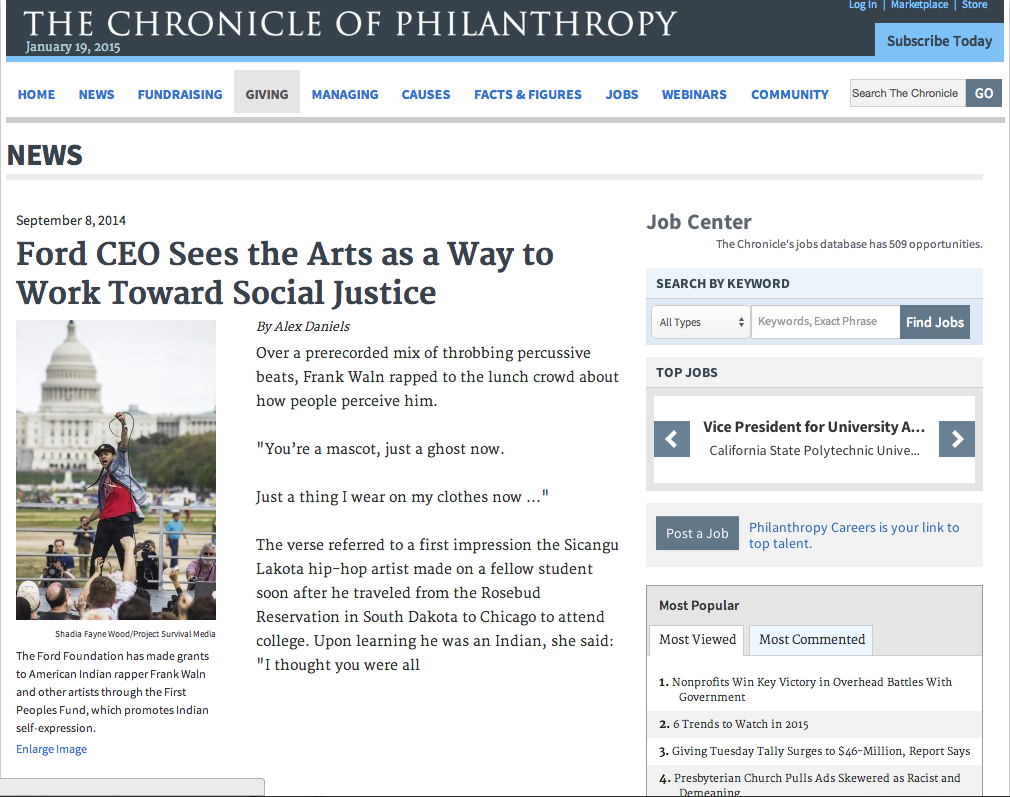This is a screenshot of The Chronicle of Philanthropy's webpage from January 19, 2015. The page features options for subscribing, logging in, and accessing their marketplace and store. On the left-hand side, there's a news article dated September 8, 2014, titled "Ford's CEO Sees the Arts as a Way to Work Towards Social Justice," written by Alex Daniels.

The article describes a scene where Frank Wallen, a Sikangu Lakota hip-hop artist, performed a rap to a lunchtime audience. Over throbbing percussive beats, Wallen rapped about societal perceptions of him, expressing sentiments like, "You're a mascot, just a ghost now, just a thing I wear on my clothes now." This verse was inspired by an interaction Wallen had shortly after moving from the Rosebud Reservation in South Dakota to attend college in Chicago. Upon learning about his Native American heritage, a fellow student remarked, "I thought you were all..."